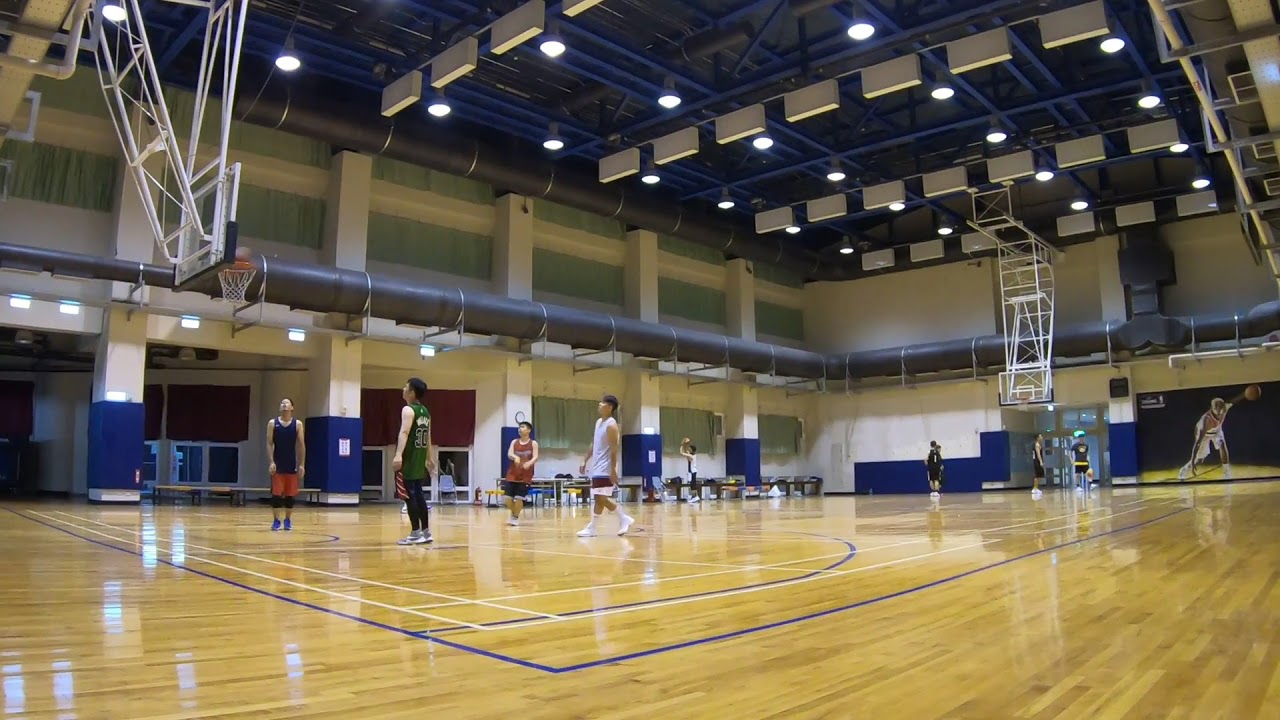The indoor basketball gym features a polished, light-colored wood floor, intricately marked with blue and white lines to denote the play area. The roof is adorned with blue-painted support pillars and beams, alongside a gray pipe running horizontally through the center. The focal point is a basketball hoop suspended from the ceiling to the left, with a basketball currently going through the net. On the left side of the image, four people look towards the hoop, including a person in a green sleeveless shirt with the number 30, black pants, a person in a blue tank top with red shorts, another in a red shirt with black shorts, and one in a white shirt with brown shorts. Further in the distance on the right side are four more individuals, all dressed in black and yellow uniforms. Centered in the image, yet off the court, is someone poised as if shooting a basketball, potentially practicing their form. Adding to the composition, a mural of a basketball player adorns the right wall, bringing the scene to life with vivid touches of orange, red, black, gray, and teal.